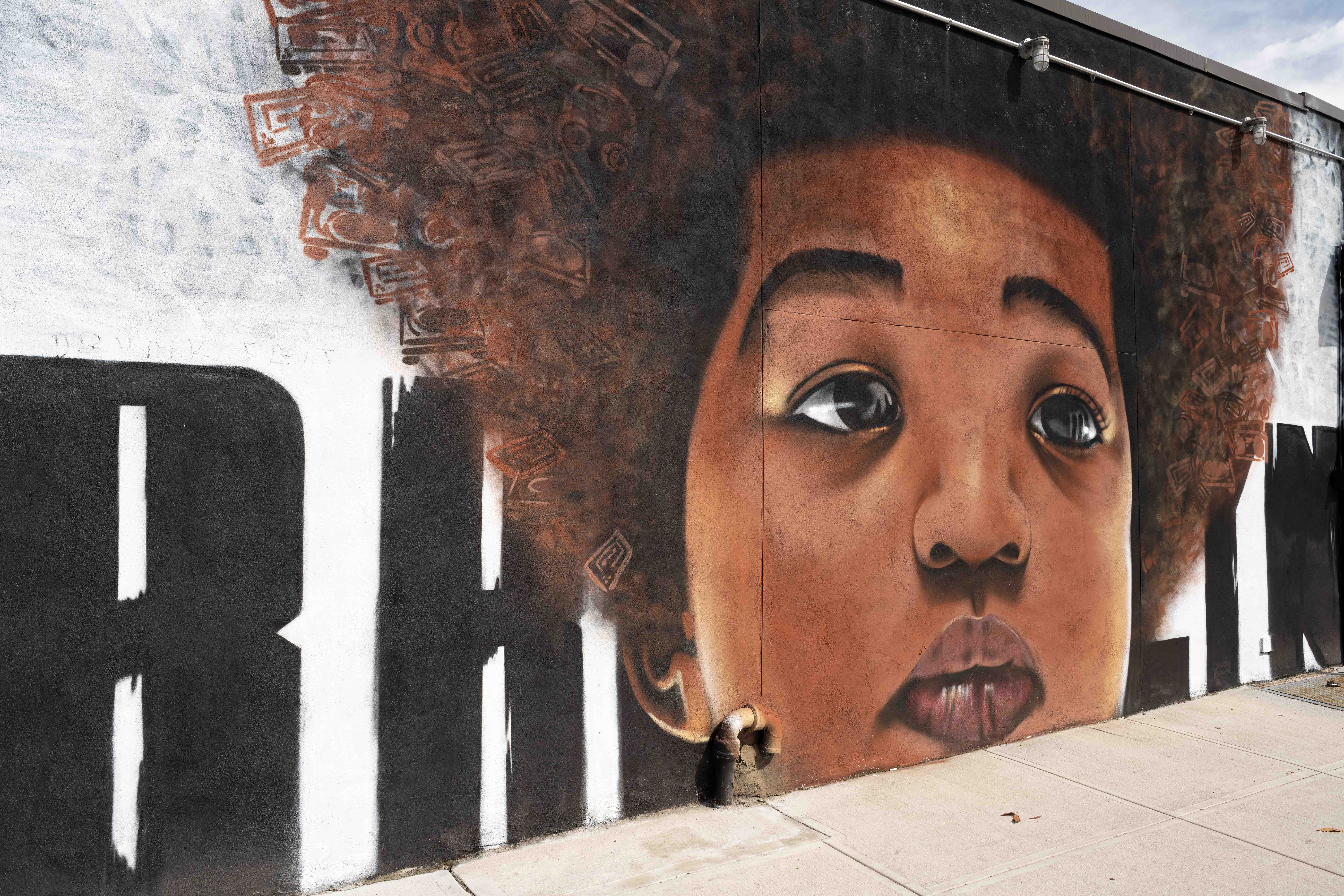In this vibrant mural, an African-American woman is depicted on the side of a building, painted with extraordinary detail. She has thick lips, brown eyes, and brown eyebrows, with her ears subtly visible. Her voluminous afro, which dominates the image, is filled with intricate etchings of musical devices such as headphones, boomboxes, portable speakers, turntables, and vintage magnetic cassettes reminiscent of the 1980s. These artistic elements suggest a possible tribute to a music icon or rapper. Behind her head, partially obscured letters spell out what looks like "BALLIN," although the full word is cut off. A pipe emerges from the ground next to the mural, mounted on the wall. The scene is set against a backdrop of a blue sky scattered with fluffy white clouds, indicating it is daytime.